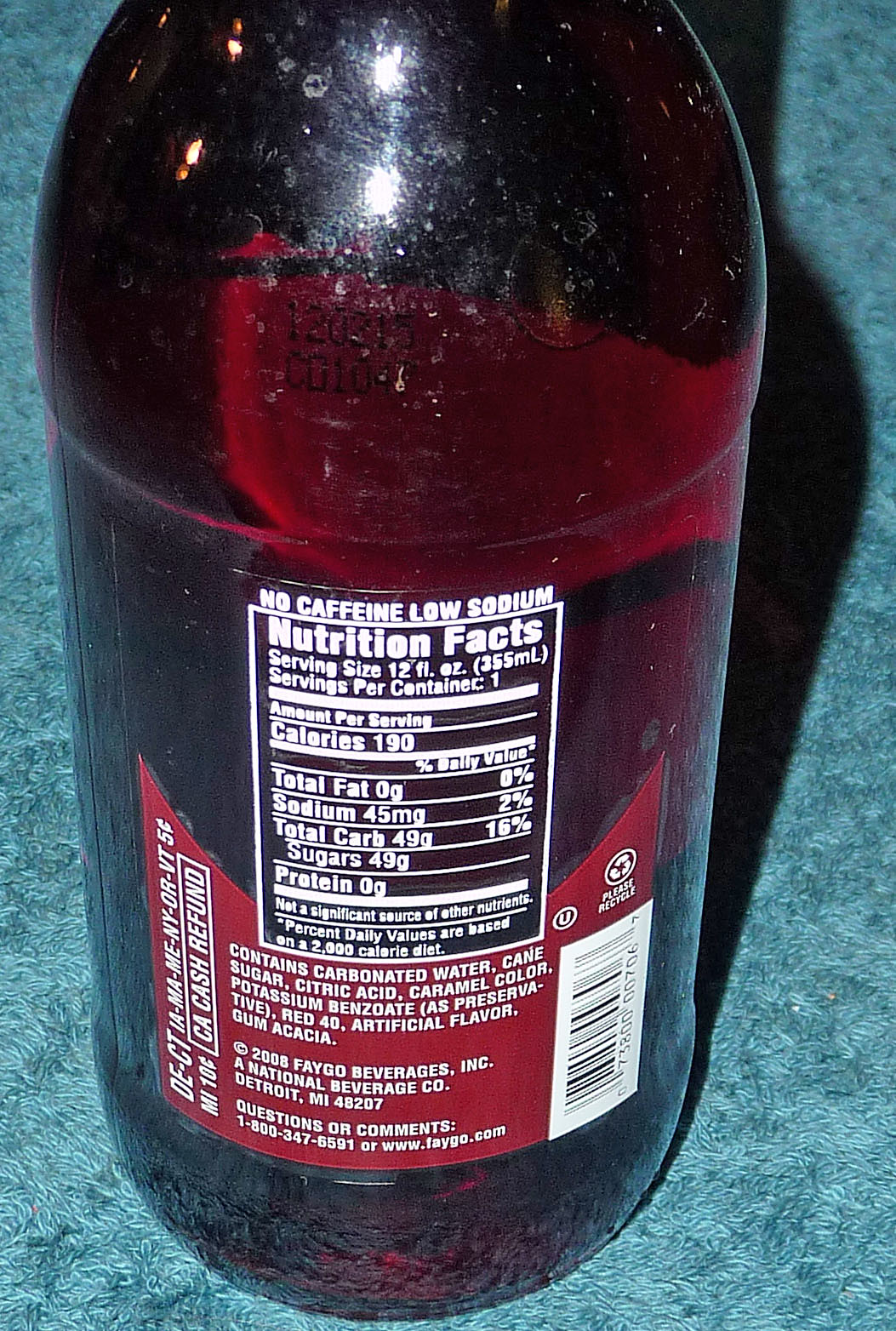The image showcases a close-up view of a plastic bottle filled with a dark red liquid, likely reminiscent of a Dr. Pepper type beverage. The bottle is positioned on a light blue surface with subtle dark blue flecks, potentially a table or carpet. The perspective captures the bottle from the back, cutting off at the neck at the top of the image and extending to the bottom edge. 

Midway down the bottle is a white nutritional label detailing the beverage's contents and nutritional information. The label prominently displays "no caffeine, low sodium" at the top. Below, it lists "Serving size: 12 fluid ounces," and provides nutritional data including "Calories: 190," "Total Fat: 0 grams," "Sodium: 45 milligrams (2% daily value)," "Total Carbs: 49 grams (16%)—all from sugars," and "Protein: 0 grams." 

Key ingredients are carbonated water, cane sugar, citric acid, caramel color, potassium benzoate (as a preservative), Red 40, artificial color, and gum acacia. The label also mentions that the product is made by Faygo Beverages, Inc., a national beverage company based in Detroit, Michigan, with a copyright date of 2008.

Flanking the nutritional facts on the left is a yellow-outlined red triangle, and below the white section of the label is a red band extending around the base of the bottle. This red label includes additional product details, such as a website link (www.faygo.com) and a contact number for customer inquiries or comments. The bottle shows slight wear with a few dings, adding to the authenticity of the everyday product depiction.